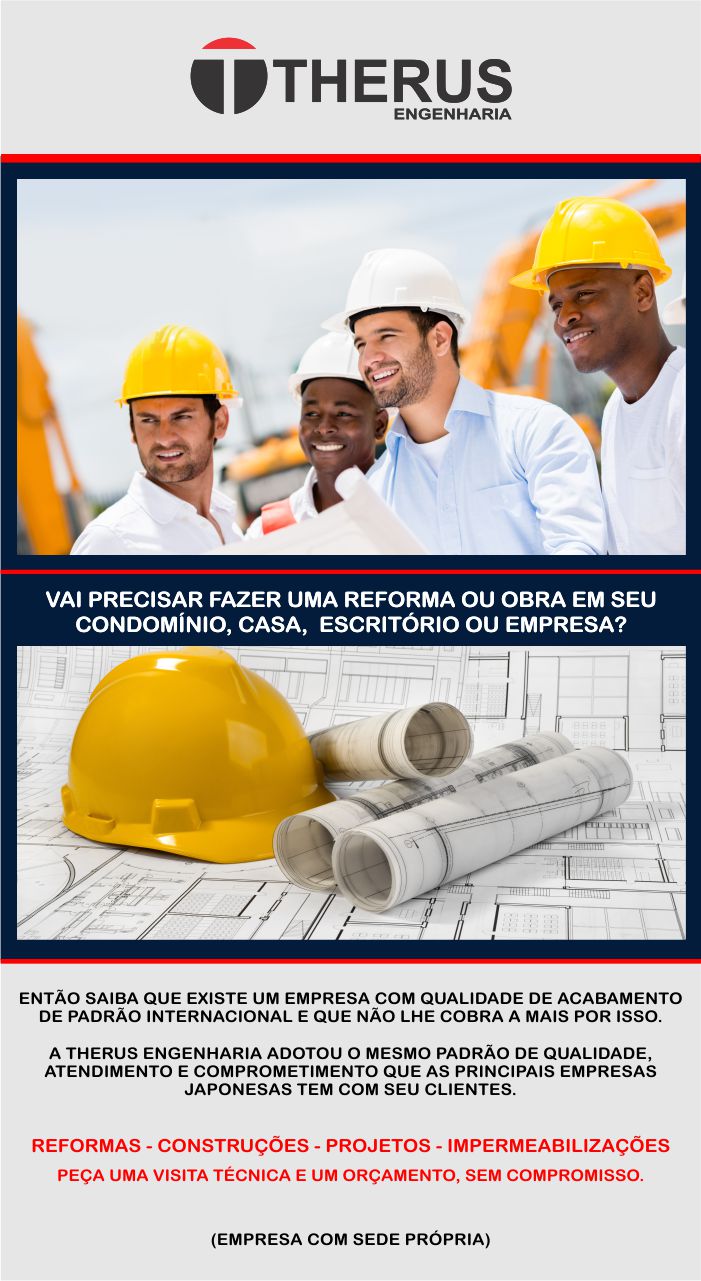This advertisement features a vertical rectangular layout with the company's logo at the top. Against a light gray background, the logo comprises "Theris" alongside a 'T' emblem on a red and black backdrop, followed by the word "ENGENHARIA." Below the logo, there is a photograph of four men, all wearing hard hats and smiling while looking to the left. They are dressed in collared button-up shirts, emphasizing a professional construction or engineering setting.

Underneath this image is a second picture showcasing a hard hat resting on a set of architectural blueprints. Some of the blueprints are laid flat, while others are rolled up, reinforcing the construction and engineering theme of the advertisement.

The bottom section of the ad contains three paragraphs of text. The first two paragraphs are written in black font, while the final paragraph stands out in red. Overall, this detailed and structured advertisement highlights the professional services offered by the company, catering to construction, renovation, or engineering projects.